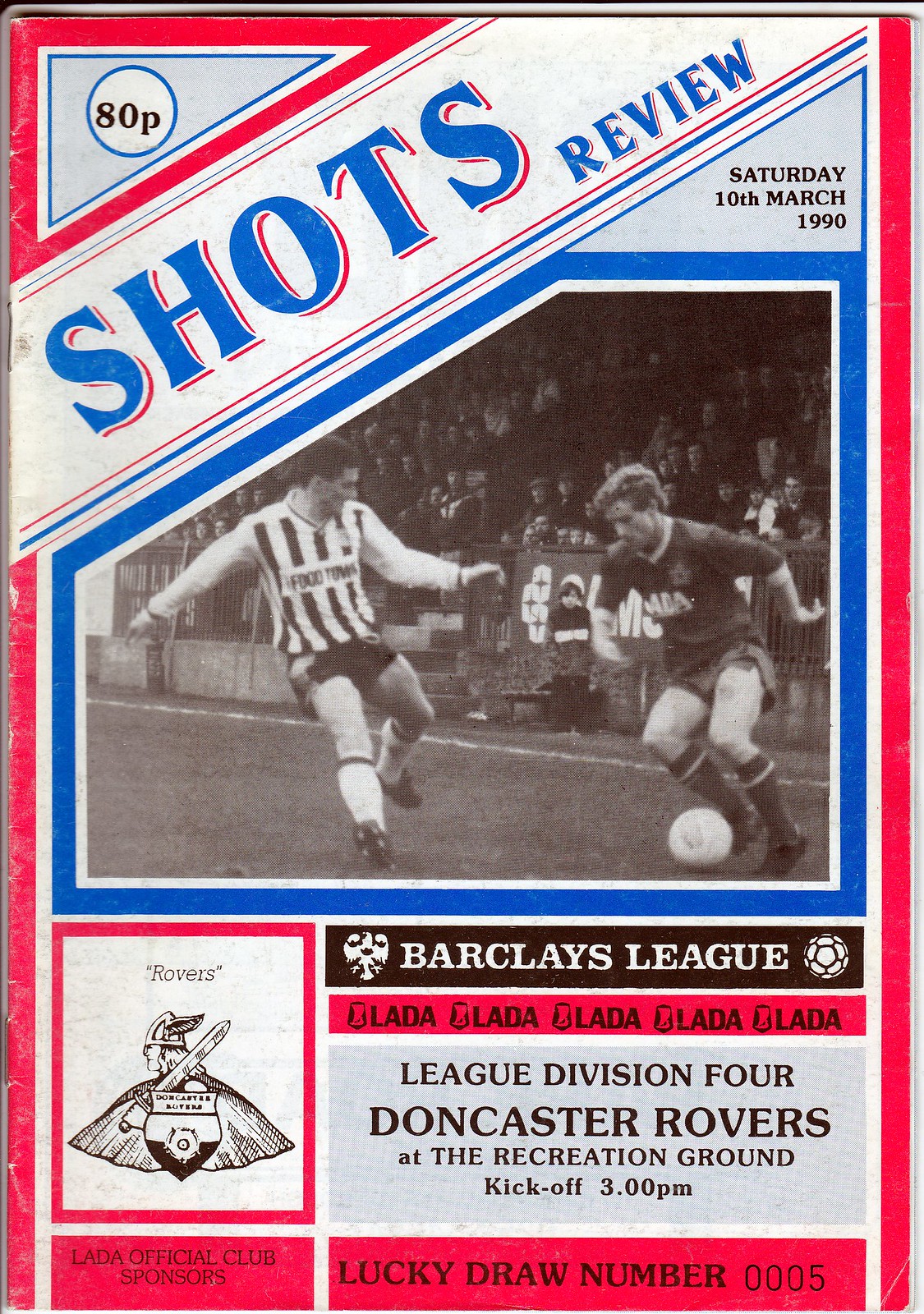This is a detailed poster from Saturday, March 10th, 1990, for a soccer match program booklet. The design features a background predominantly in red with white triangles. At the top, in the upper left, it says "ADP." Below that, running diagonally upwards in blue lettering with a red outline, it reads "Shots Review." The main focal point is a black and white image of two Caucasian soccer players on the field, one preparing to kick the ball. Beneath the image, it states "Barclays League, League Division Four, Doncaster Rovers at the Recreation Ground," with a kickoff time of 3 p.m. Additionally, there's a "Lucky Draw" number displayed as 0005. Adjacent to this, underneath the black and white photo, there is an illustration design featuring the word "Rovers" and what appears to be a Viking or figure with a sword. To complement this, an emblem or shield signifies "Lada Official Club Sponsors."